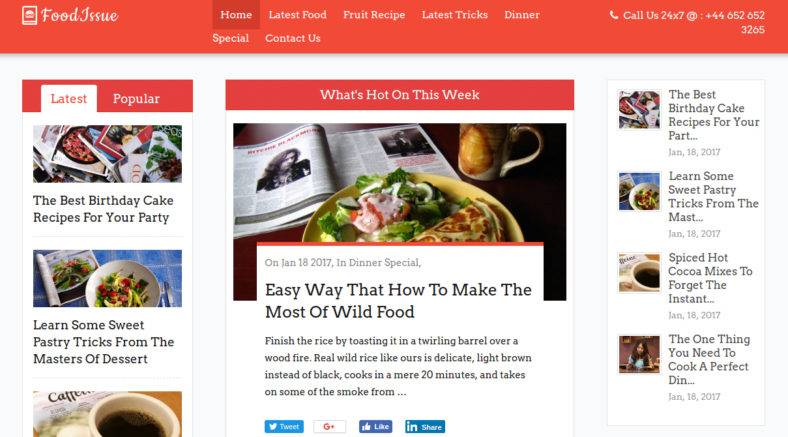This is a detailed descriptive caption for the provided image:

---

Screenshot of the Food Issue website homepage. 

**Top Left**: The site’s logo, 'Food Issue,' accompanied by an icon resembling an open book, symbolizing a virtual magazine.

**Navigation Bar**: Positioned at the top with several tabs. The 'Home' tab is highlighted in a darker shade, indicating it is the currently selected section. Additional tabs include:
- Latest Food
- Fruit Recipes
- Latest Tricks
- Dinner Specials
- Contact Us

**Top Right**: A call link reads, "Call us 24/7 at 446-526-523-265."

**Main Content**:
- **Left Sidebar**: Displays the latest articles in a vertical list:
  1. "The Best Birthday Cake Recipes for Your Party"
  2. "Learn Some Sweet Pastry Tricks from the Masters of Dessert"

- **Center Section**: Features the headline "What's Hot This Week" with a main article titled "Easy Way to Make the Most of Wild Food". Note: The title's grammar appears unusual.

This layout and content organization provide an engaging overview of the culinary articles and resources available on the Food Issue website.